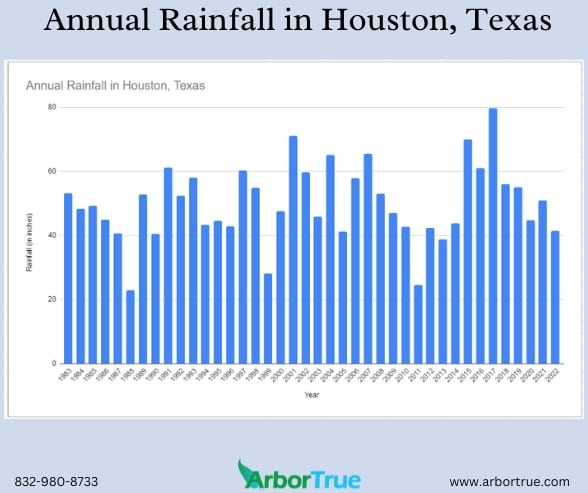The image features a detailed bar graph titled "Annual Rainfall in Houston, Texas," set against a light blue background. The x-axis spans from 1983 to 2022, while the y-axis measures rainfall in inches, with increments marked at 0, 20, 40, 60, and 80. The bars, colored blue, show fluctuating rainfall patterns over the years, indicating several peaks and troughs. At the bottom of the graph, contact details are provided: "832-980-8733" on the left corner, "Arbor True" in green and blue text in the center, and the website "www.arbortrue.com" on the right. The graph appears to represent data likely from an Arbor True presentation.